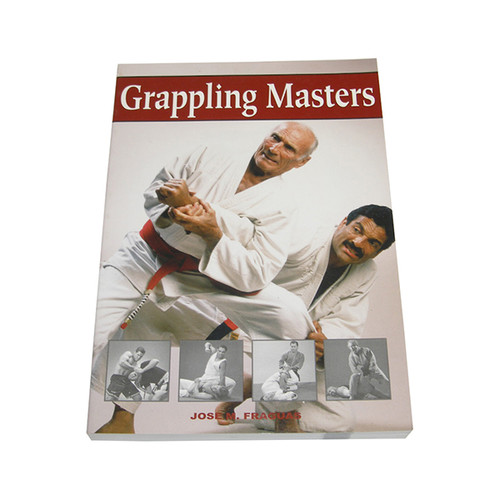The magazine cover features a dynamic martial arts scene set against a plain white background. Dominating the image are two individuals in white martial arts uniforms. Both men are engaged in a grappling technique. In the foreground is an elderly, vigorous white man who is bald with a fringe of white hair. He is wearing a red belt and adopting a wide stance with his legs spread and feet firmly planted on the ground, his posture showcasing his experience and strength. The elder is grabbing the wrist of the second man, a darker-skinned individual with thick black hair and a prominent mustache. The younger man appears to be struggling to free his arm, even attempting to pull on the elder's pants with his left hand to destabilize him. Above this intense scene, a red banner stretches across the top of the cover with bold white text that reads "Grappling Masters." At the bottom of the cover, four smaller black-and-white photographs are superimposed, depicting various martial arts techniques, including neck grabs, ground control, and defensive maneuvers. Below these action shots, although partly obscured and challenging to read, the text appears to proclaim "Joseph Fraouaz."